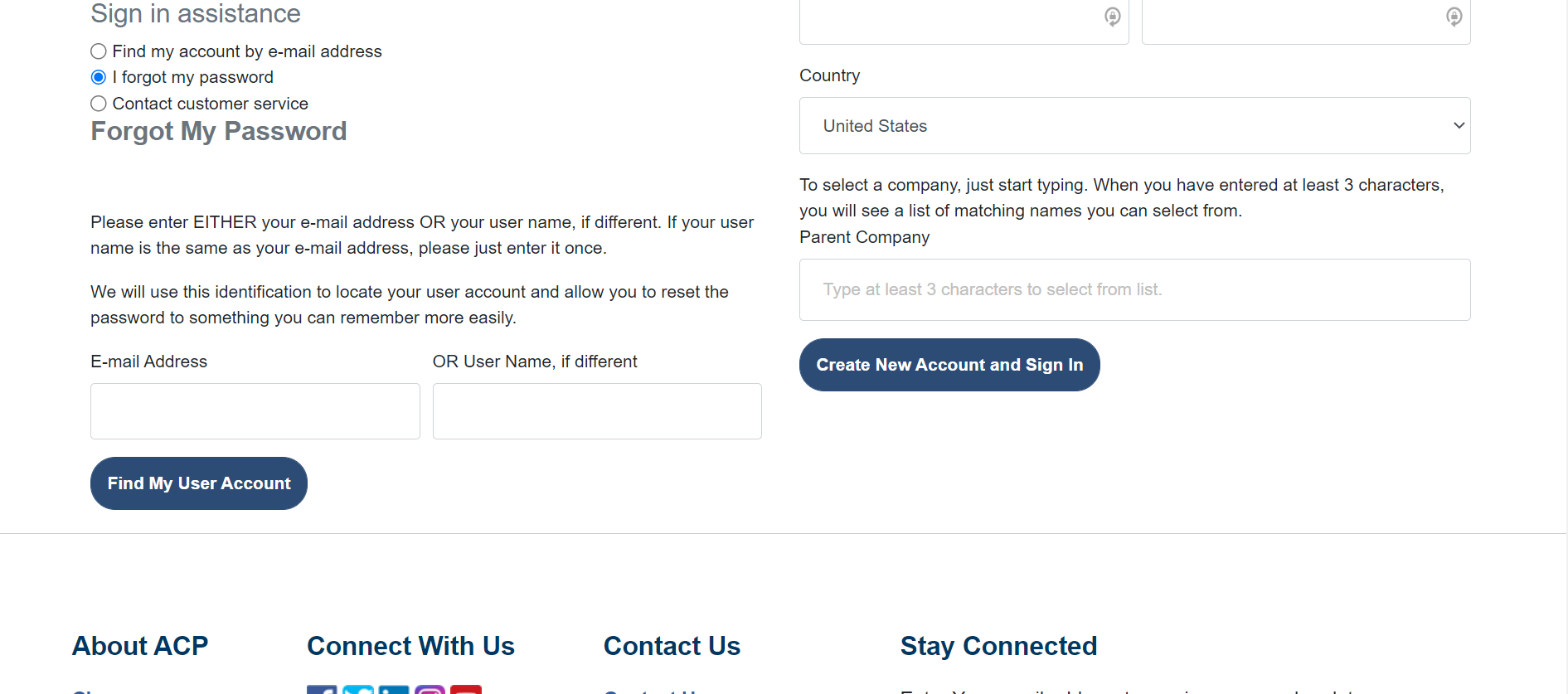The image portrays a "Forgot Password" page designed to assist users in recovering access to their accounts. At the top of the page, users are instructed to either enter their email address or username. A note clarifies that if the username is the same as the email, users should only enter it once. Below this instruction is a text field where users can input their email or username.

The page features three radio button options to further aid in account recovery: "Find my account by email address," "I forgot my password," and "Contact customer service," with the "I forgot my password" option pre-selected. The form also includes a drop-down menu on the right side for users to select their country, defaulting to the "United States."

At the bottom of the form, two prominent dark navy blue buttons are visible. The first button, labeled "Find My User Account," allows users to proceed with account recovery. The second button, labeled "Create New Account and Sign In," offers an alternative option for those who may want to set up a new profile.

The partially visible footer suggests a well-structured page layout, although its details are cut off in the image.